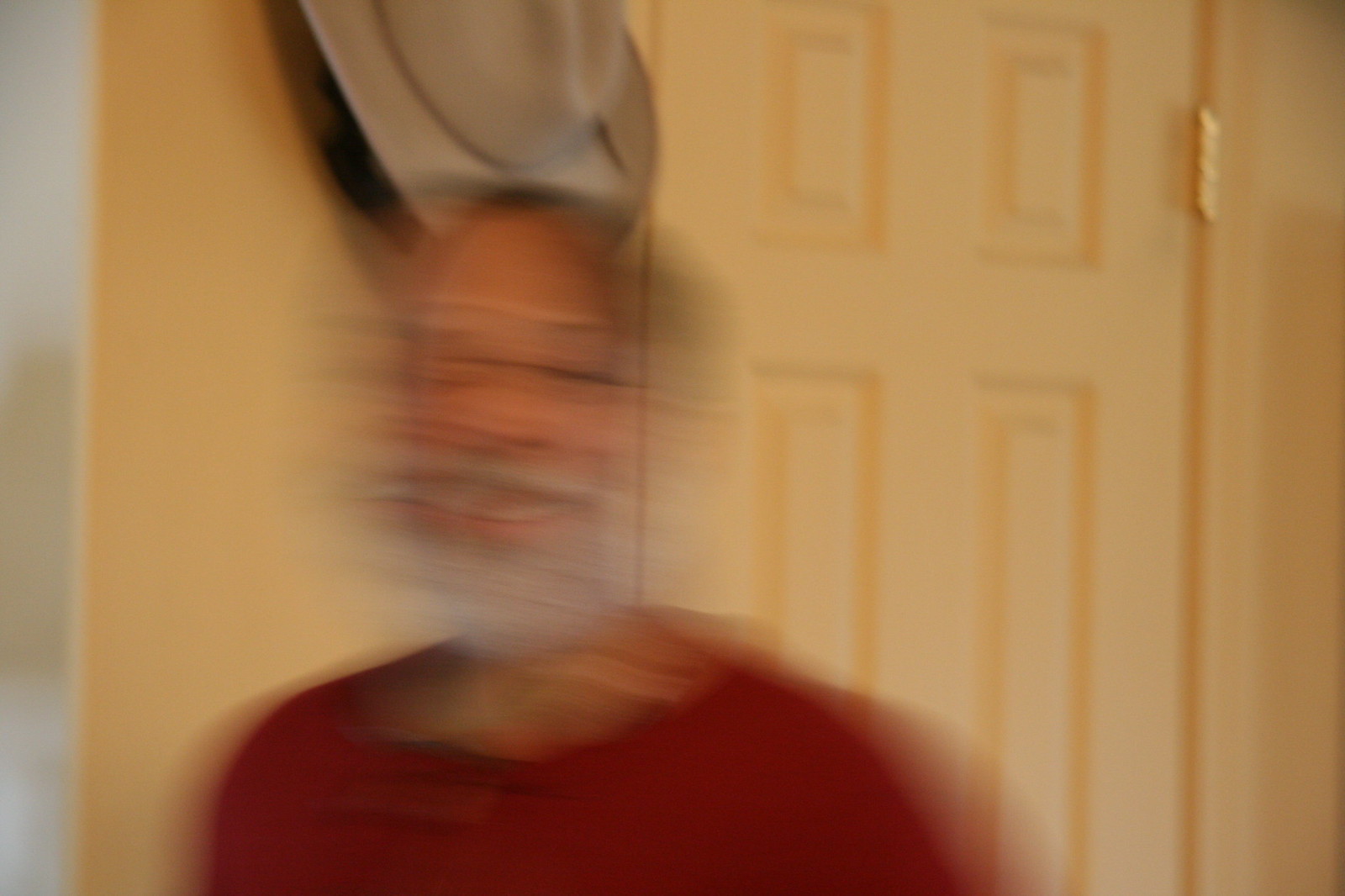In this blurry, out-of-focus photograph, a man stands smiling against a softly colored background. The wall behind him appears to be a delicate shade of either soft yellow or off-white. Prominently visible is a door with gold hinges, sporting two short indented rectangles at the top and two elongated ones at the bottom. To the left hangs a tan cowboy hat, adding a rustic touch to the scene. The man, who seems to be either bald or sporting very short dark hair, radiates warmth with his smile. His facial hair—a mustache and beard—has turned gray or white, contrasting with his bright red, collarless shirt. The overall composition exudes a sense of casual, understated charm.